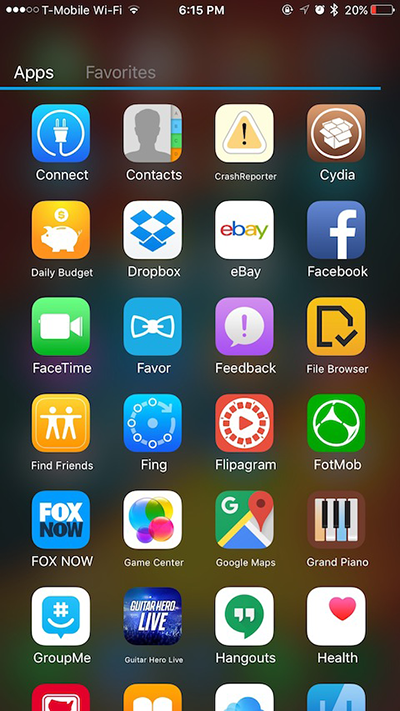This image captures the front screen of a cell phone with intricate details. In the top left corner, a network status indicator shows four filled white dots alongside four unfilled ones, right next to the "T-Mobile Wi-Fi" network label. The time displayed is 6:15 PM. Several icons are visible on the status bar, including a clock, Bluetooth symbol, and a battery icon showing 20% remaining charge.

The screen heading features two labels: "App," rendered in white, indicating it is the active selection, and "Favors," in green, showing it is not currently selected. Beneath the "App" label runs a distinct blue line.

The screen is organized into seven rows of app icons, each row containing four apps. Due to the screen cutoff, the names of the apps in the bottom row are not fully visible. Starting from the top row and moving left to right, the apps are:

1. **Connect**
2. **Contacts**
3. **Crash Reporter**
4. **Cydia** (noted with the spelling CYDIA)

In the second row:

5. **Daily Budget**
6. **Dropbox**
7. **eBay**
8. **Facebook**

In the third row:

9. **FaceTime**
10. **Favor**
11. **Feedback**
12. **File Browser**

In the fourth row:

13. **Find Friends**
14. **Fing**
15. **Flipagram**
16. **FotMob** (noted with the spelling FOTMOB)

In the fifth row:

17. **Fox Now**
18. **Game Center**
19. **Google Maps**
20. **Grand Piano**

In the sixth row:

21. **GroupMe**
22. **Guitar Hero Live**
23. **Hangouts**
24. **Health**

Due to the bottom row being cut off, the names of the final four apps are not visible. The background of the screen is blurred and multicolored, making it hard to discern any specific details or patterns.